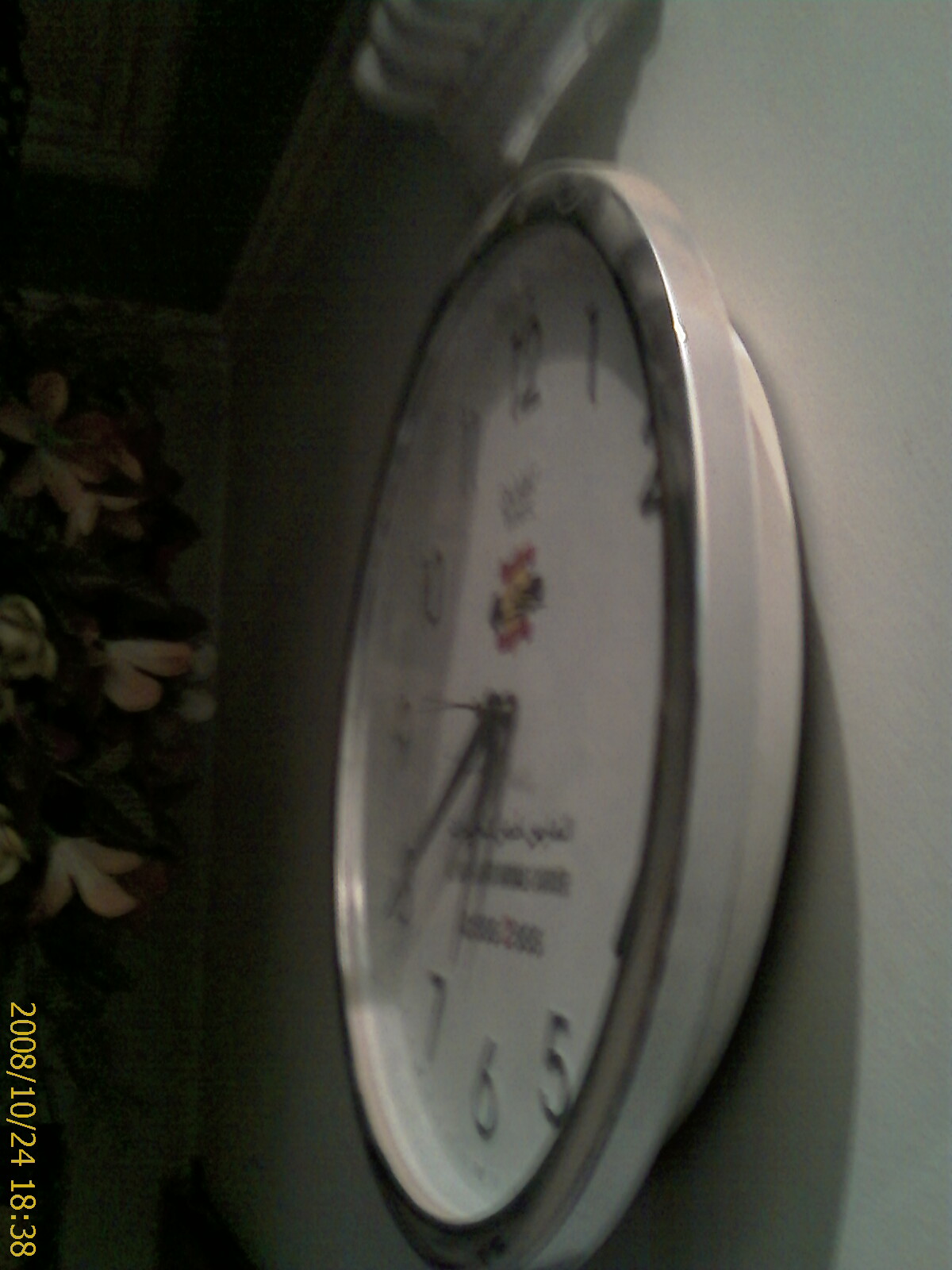This close-up side view of a wall-mounted clock captures its classic design, albeit in a somewhat blurry image that obscures finer details. The clock features a round metallic rim, likely made of silver or chrome, contributing to its timeless and simple appeal. The clock face is pristine white, with bold black numbers marking the hours in a straightforward, unadorned font. The hands of the clock are slender and black, maintaining the clock's minimalist aesthetic. Near the center of the face, there's a small, colorful design or logo, although the blurriness of the photo makes it difficult to discern the specifics of this decoration. This subtle yet charming element introduces a hint of personality to an otherwise functional and utilitarian item.